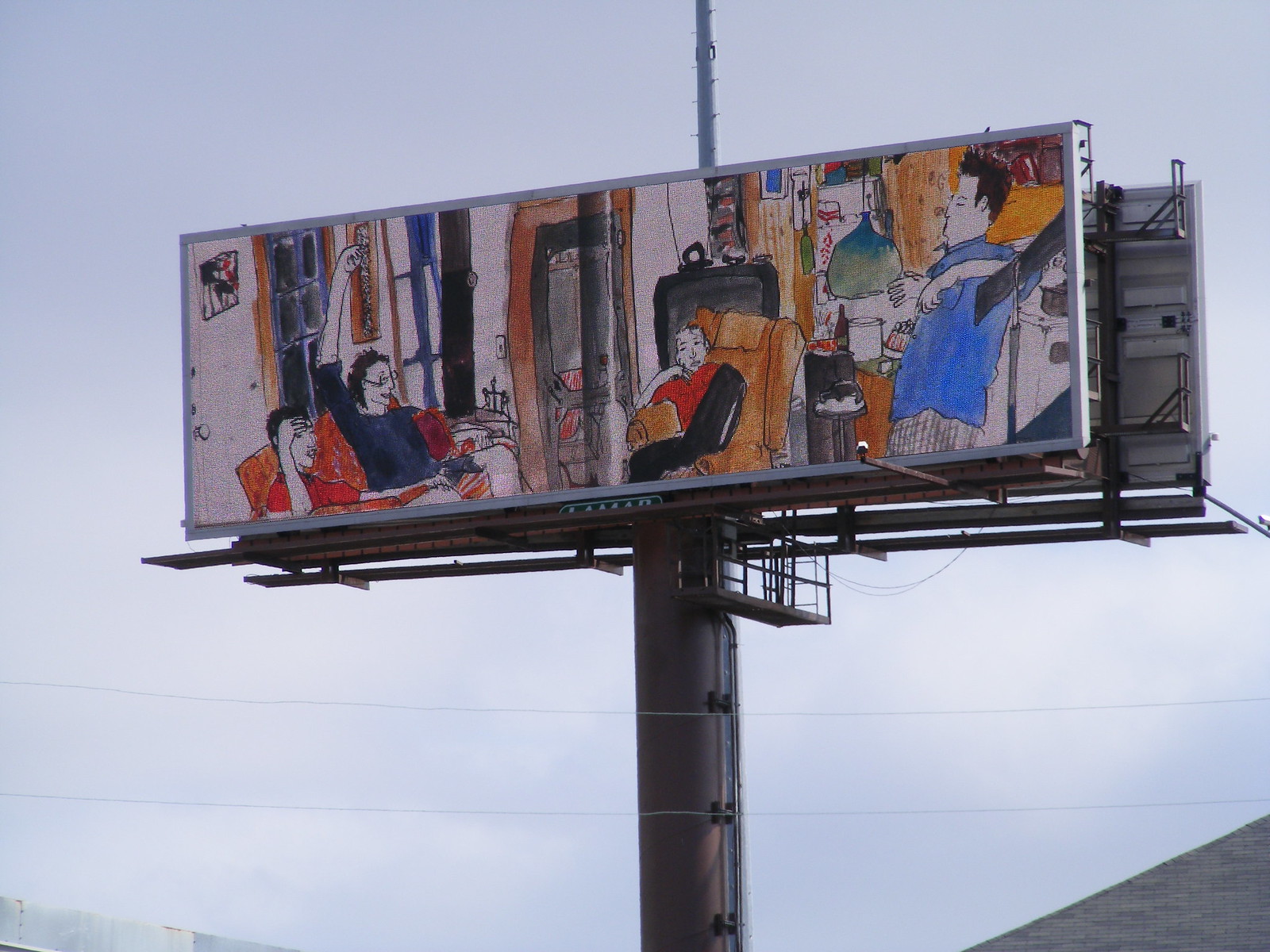The image features a detailed billboard illustration depicting a lively scene of friends hanging out in an apartment. The rectangular sign, which is mounted on a thick brown pole, is outlined in gray. The scene captures two friends seated on an orange sofa; the friend on the left is wearing a blue shirt with his arm raised, while the friend on the right sports a red shirt. To their right, another individual sits on a brown chair, dressed in a red shirt and black pants. Further to the right, a friend with spiky black hair and a blue shirt is leaning against something. The bottom right corner of the image reveals a gray rooftop in the background. Additionally, adjacent to the primary billboard, the back portion of another sign is visible on the right. The sky in the backdrop is a uniform light blue, adding to the pleasant ambiance of the scene.